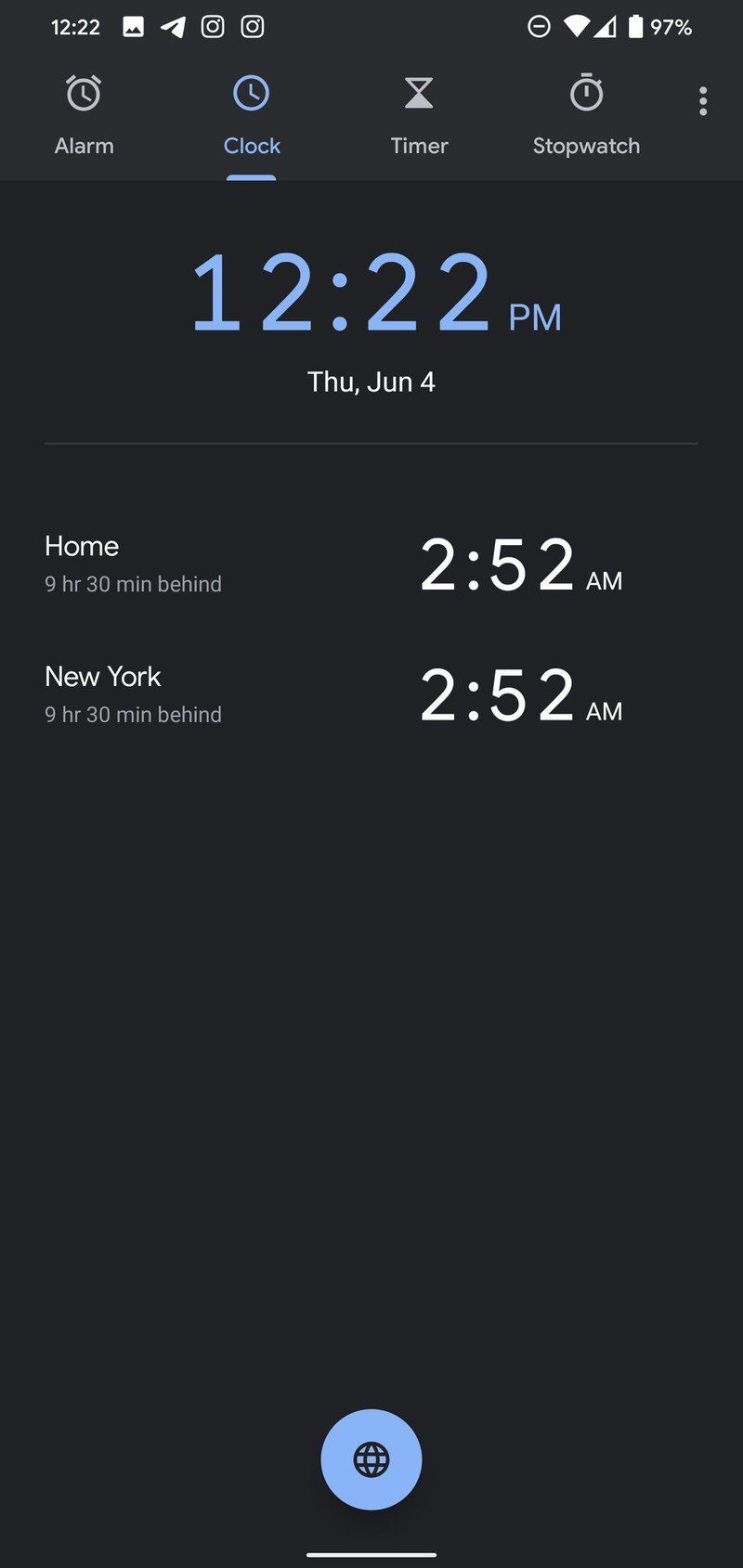This is a detailed and cleaned-up descriptive caption for the given image:

---

The screenshot on the phone displays a time of 12:22 in the top left corner. Next to it, on the right, there are several icons: a gallery icon, an arrow, and two Instagram icons. Further to the right, there is a circle with a minus sign in the middle, a Wi-Fi symbol, and three-quarters full signal bars arranged in a triangle shape. Additionally, a white battery symbol indicates a charge of 97%. 

Below these icons, the screen shows the word "Alarm" with a white alarm clock icon. Next to it, there's a clock with a blue highlight, followed by "Timer" accompanied by a white sand timer icon, and "Stopwatch" with a stopwatch icon. Beneath these, three white dots are aligned vertically.

The time "12:22 p.m." is displayed in blue, matching the clock highlight, and beneath it, "Thursday, June 4th" is written in white text. A thin white line separates this section from the next.

The screen then shows "Home" with the note "9 hours 30 minutes behind" alongside a time of "2:52 a.m." in white text. Similarly, "New York" with the same time difference and time is displayed below "Home."

At the very bottom, there's a light blue circle with a black globe icon in the center, and a small white line beneath it. The background of the screenshot is primarily dark black, with the top portion being a lighter shade of black.

---